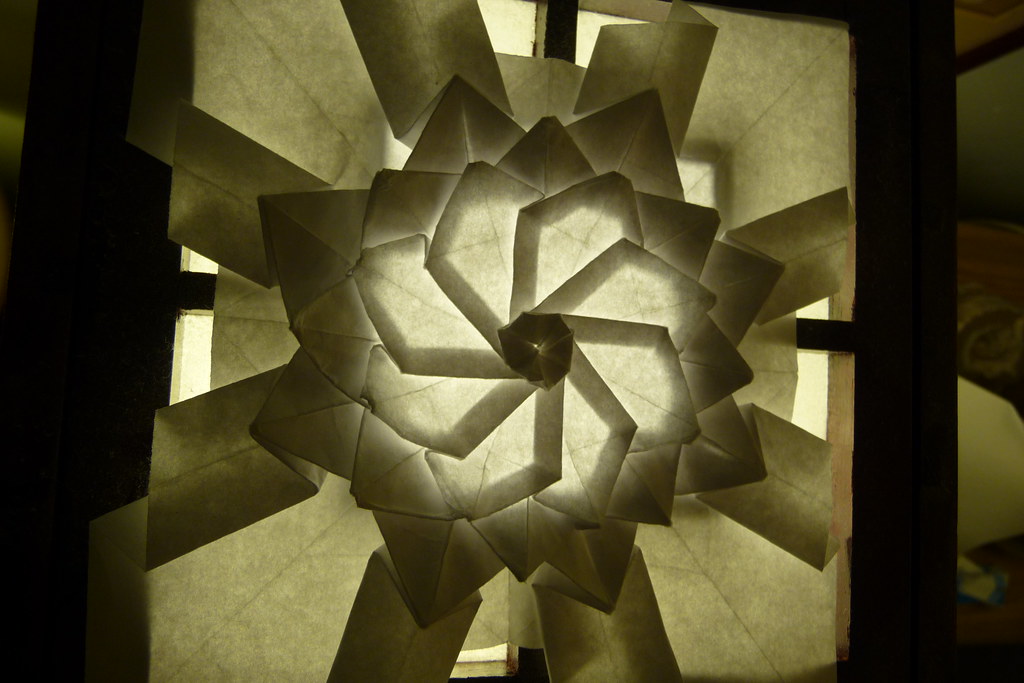The photograph captures an upward view from the ground, looking towards the peak of a ceiling, likely a dome. Central to the image is a highly detailed, concentric, flower-like structure with multiple layers, creating a three-dimensional effect. The petals, which have a resemblance to kites or fan paddles, are arranged in various layers: the inner-most layer has six or seven smaller petals, followed by a middle layer of slightly larger petals, and an outer layer with seven or eight long, thin strips. These layered petals are illuminated by light, giving the impression of a delicate, paper-thin material. The surrounding area is framed by wooden slats, possibly part of a window or structural frame, through which soft, diffuse lighting filters through, hinting at natural light from outside. The overall effect is a harmonious blend of natural and artificial elements, creating a serene and intricate play of light and shadow.